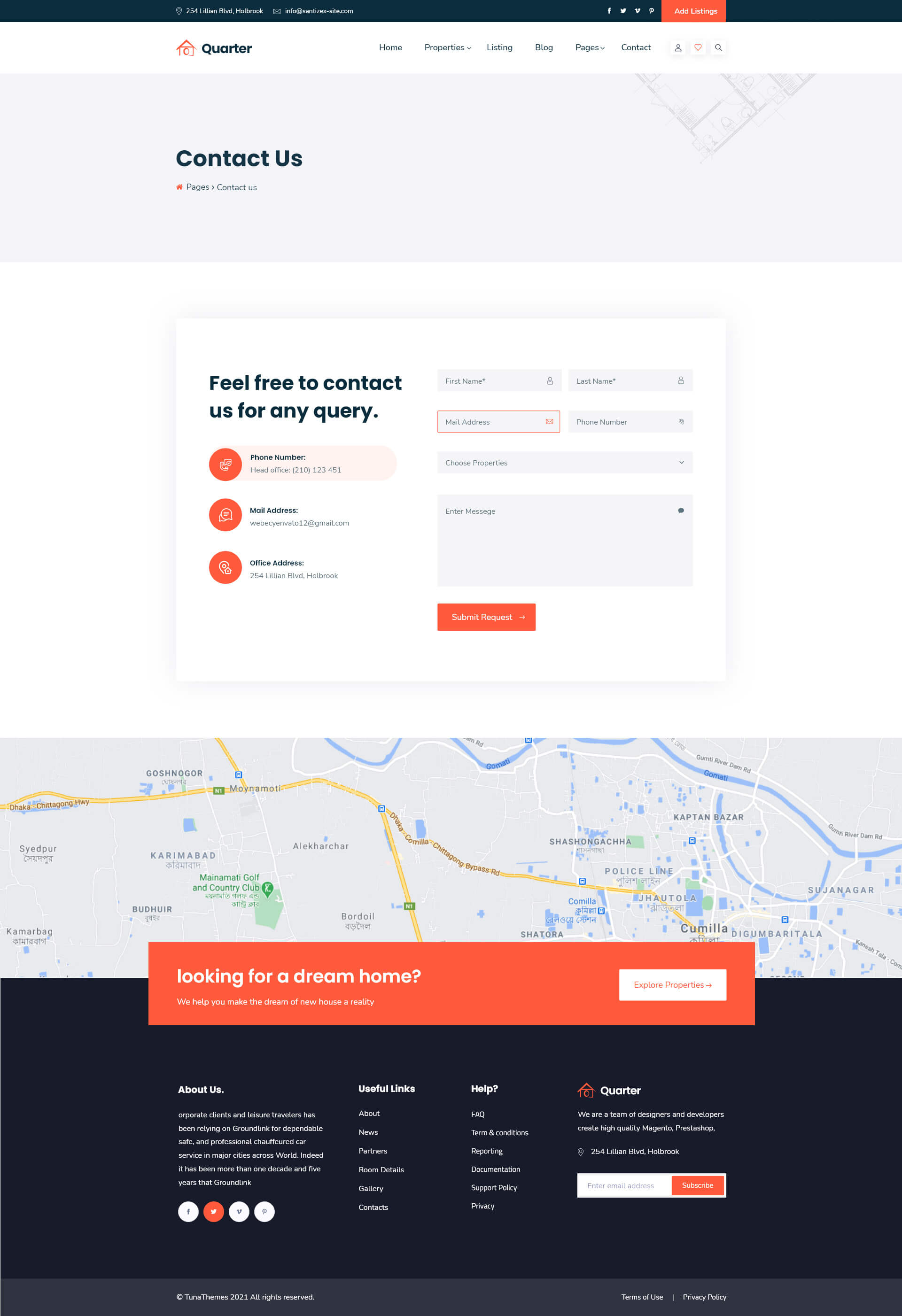This image is a detailed screenshot of a computer interface pertaining to a real estate website. In the upper left corner, there's an orange, drawing-like illustration of a house adjacent to the text "Quarter." The navigation bar underneath features several clickable options, with "Add Listings" highlighted in orange, indicating it has been selected. 

Dominating the central area of the screen is a large gray rectangle labeled "Contact Us" with smaller text underneath reading "Pages, Contact Us." A white box within this gray area contains black text stating, "Feel free to contact us for any query." Among the contact options, the phone number field is prominently marked with an orange circle, while the mail address field is outlined in orange, suggesting it has been interacted with.

In the lower third of the image, a map is visible at the top. Beneath that, an orange rectangle centered on the screen contains white text that reads, "Looking for a dream home? We help you make the dream of a new house a reality." To the right of this, a white box invites users to "Explore Properties."

The bottommost section features a black background with additional information about "The Quarter Company." This area includes sections labeled "About Us," "Useful Links," and "Help," providing further resources and company details.